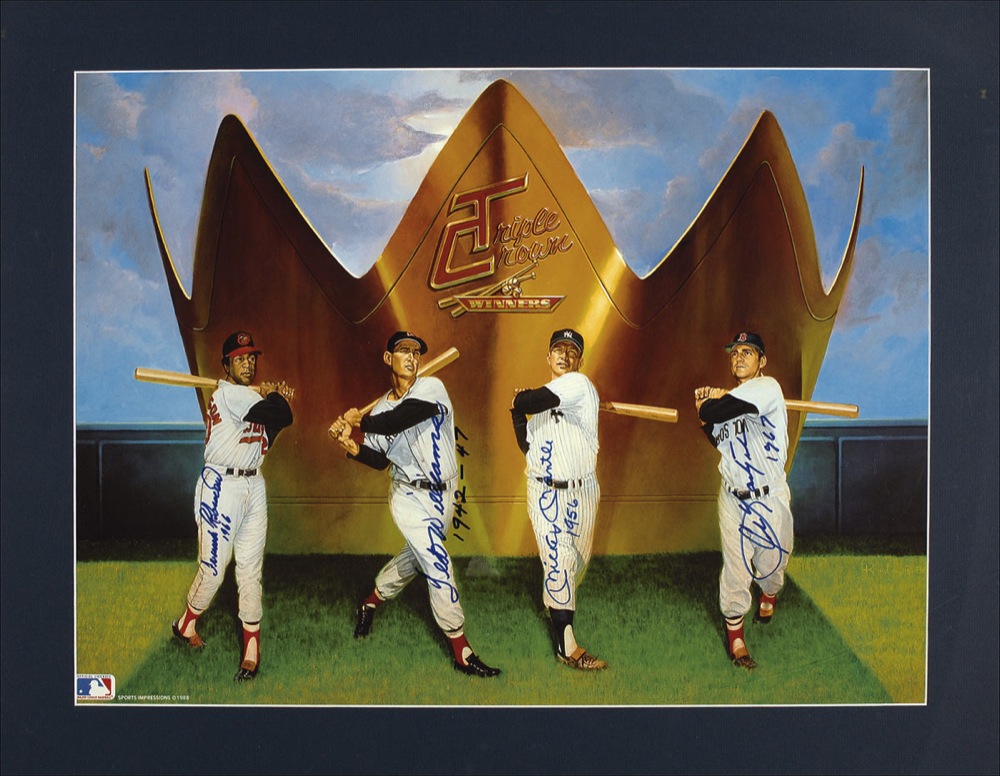The image is a rectangular, framed commemorative painting capturing a realistic depiction of four legendary baseball players standing on a bright green turf field. Centered in the background is a large, shiny golden crown with the prominent letters "C" and "T" in a stylized format, with additional cursive writing in red that reads "Triple Crown Winners." Beneath these letters, there is the word "Winners" clearly inscribed. 

The four players, standing roughly centered, are positioned as follows from left to right:
1. A dark-skinned man in a black hat, wearing a white and red baseball shirt and white socks, holding a bat behind him.
2. A lighter-skinned man donning a white baseball ensemble, also with a bat held behind him.
3. A man dressed in a white and black striped baseball outfit, sporting a dark-colored hat, with his bat poised to swing.
4. Another man in a similar white and black striped outfit and black hat, holding a bat similarly.

In the lower left corner of the image, a Major League Baseball icon is visible, suggesting it might be a limited edition piece of baseball memorabilia. The background showcases a bright blue sky with a few white clouds, framed by a dark navy border. This piece also appears to include autographs and dates associated with each prominent player, celebrating their achievements as Triple Crown winners.